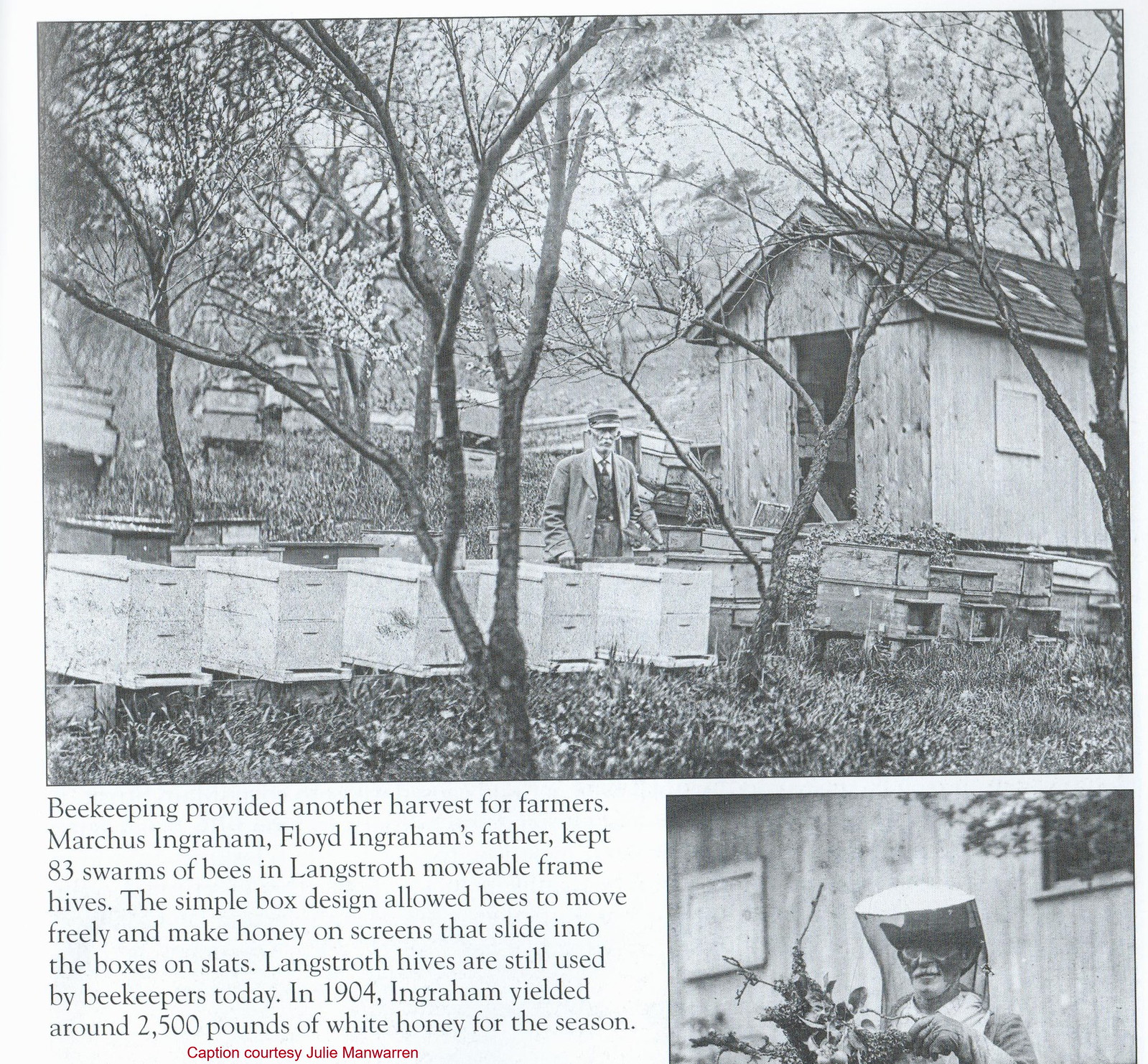The black and white image, occupying three-quarters of this square frame, captures an old man with a suit, hat, beard, mustache, and white hair, exuding a refined, 19th-century formal style. He stands next to several wooden beekeeping boxes in what appears to be a backyard with a shed to his right, scattered long grass, and flowering trees in the background. Accompanying the main image is a smaller, rectangular inset in the bottom right. This secondary photo features the same man, Marcus Ingraham, wearing an old-fashioned beekeeper's net over his face and holding twigs and branches, likely engaged in beekeeping activities. The text to the left of the inset provides historical context, explaining that Marcus Ingraham, Floyd Ingraham's father, managed 83 swarms of bees in Langstroth movable frame hives around 1904, yielding approximately 2,500 pounds of white honey for the season. The Langstroth hives allowed bees to move freely and produce honey on screens that slid into the boxes on slats, a design still used by beekeepers today. The caption details, provided by Julie Mann Warren, emphasize how beekeeping offered an additional harvest for farmers.